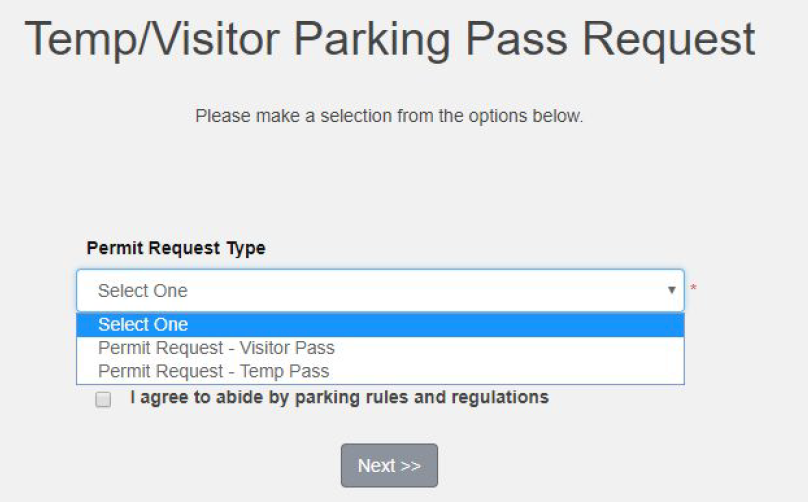The image captures a digital interface for requesting a parking pass, specifically titled "Temp/Visitor Parking Pass Request." At the top, the title is prominently displayed, followed by a smaller header instructing users to "Please make a selection from the options below." Below this, a large blank space emphasizes the formality and importance of the next steps.

The "Permit Request Type" section appears next, urging users to "Select One" in bold white text against a blue background. Within this section, users have two options: "Permit Request - Visitor Pass" and "Permit Request - Temp Pass." These selections are neatly contained within a distinct rectangular area.

Outside and below this rectangle, there is a noticeable gray box featuring an affirmation statement, "I agree to abide by parking rules and regulations," which is presumably a checkbox. Finally, at the bottom of the page, a gray button labeled "Next" with two right-pointing arrows invites users to proceed to the next step in the process.